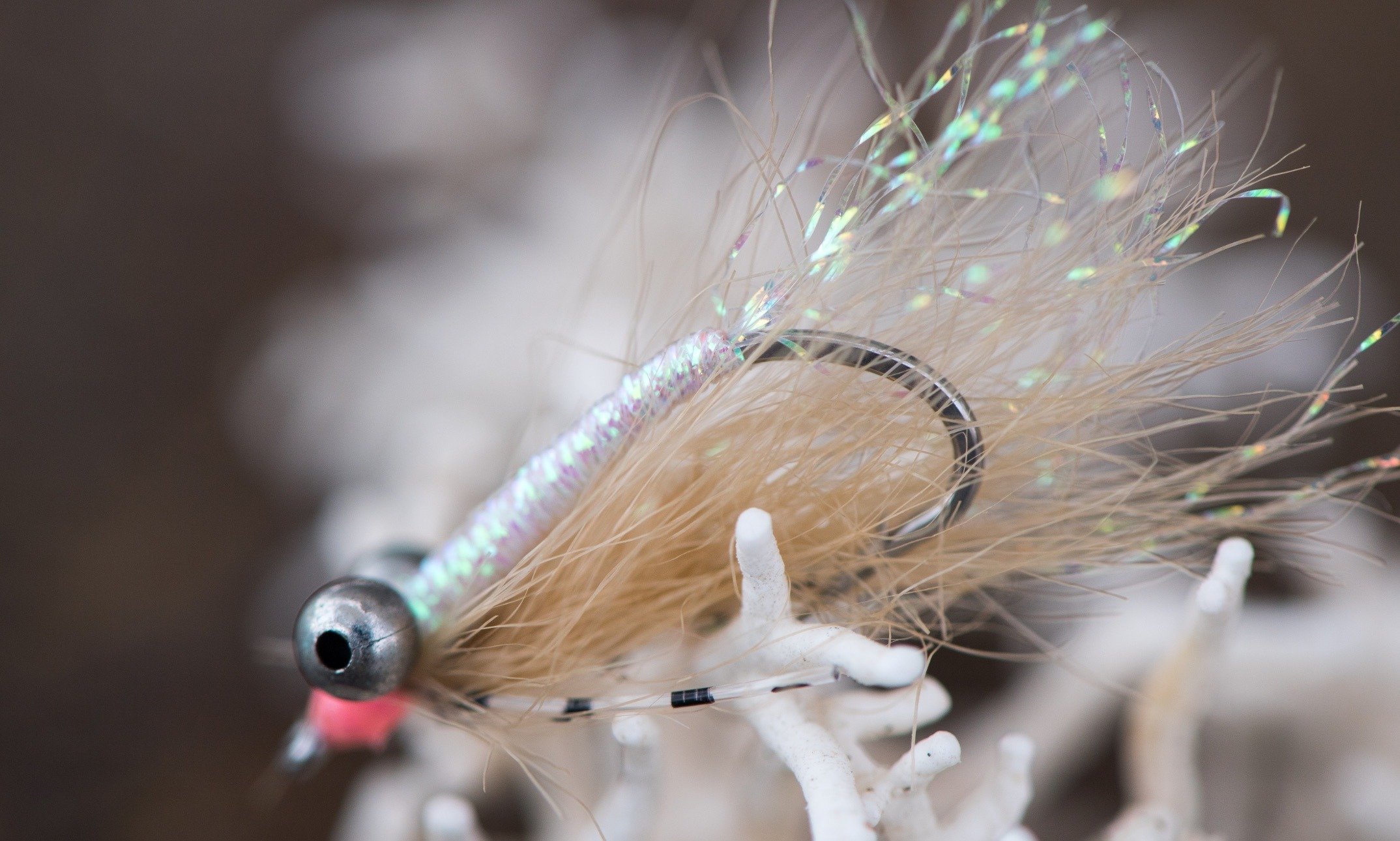This is a highly detailed close-up image of a handcrafted fly-fishing lure. The lure itself features a black gunmetal-colored steel hook, intricately wrapped with iridescent fiber that extends from the shank up to the curve of the hook. At the top of the hook, there are metallic beads serving as eyes, giving the impression of a living creature. The head of the lure includes a small red element, likely serving as a nose. Below the eyes, fuzzy material resembling dog hair or synthetic fur is attached, flowing backward and enhancing the insect-like appearance. The lure seems to be situated on or held by something spiky and white, resembling coral, though the background remains blurred and indistinct. This fly, with its detailed craftsmanship, is designed for fly-fishing, intended to mimic a prey creature to attract fish.